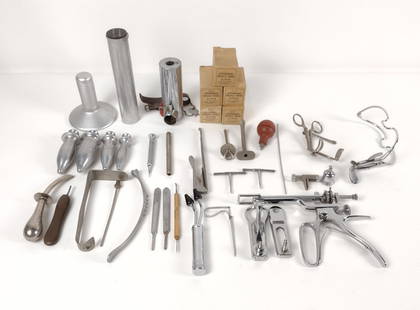The photograph captures an array of tools meticulously arranged on a white floor, possibly a countertop, against a white wall. Predominantly metallic silver or chrome in color, the collection spans several rows and consists of a variety of implements.  Hacksaws, regular saws, and large screws lie in neat rows, with some tools featuring darker wooden handles. Scattered among these are cylindrical objects and items resembling elongated plugs or perhaps antique medical instruments, such as an old-time syringe or forceps. Noteworthy are the metallic items that look like bullets situated above the hacksaws. Interspersed within the layout, dark brown cardboard boxes are stacked, adding a touch of color contrast to the scene. The overall appearance of the assemblage, with its mix of shiny metallic tools and wooden elements, evokes a sense of vintage surgical or woodworking equipment.